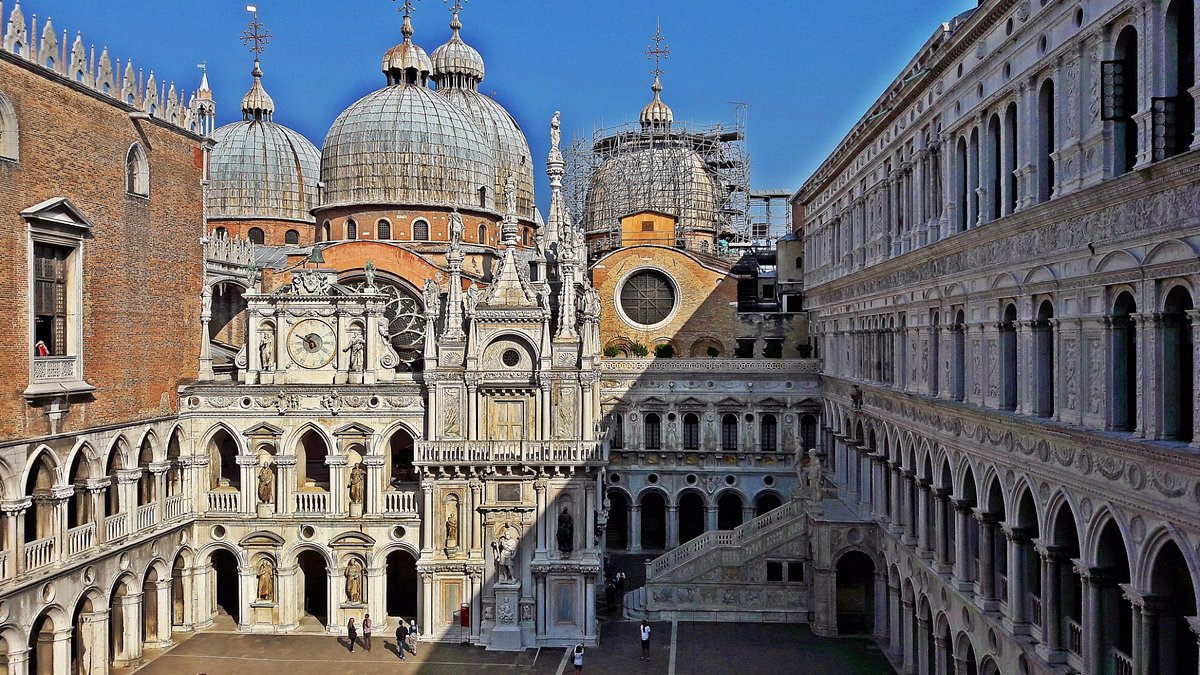The photograph captures a grand and intricate historical architectural complex, likely from medieval times. Predominantly, the structure resembles a cathedral or basilica, featuring multiple large domes topped with crosses, signaling its religious significance. The architecture is characterized by numerous archways spanning across four floors, with some portions constructed from white to light gray stone and others from red brick. The left side of the building has a more extensive brick facade, while the right side has arches on the first and second floors and casts a substantial shadow due to the sunlight illuminating the central and left portions of the square. The bright and clear afternoon sky enhances the ornate and awe-inspiring details, such as elaborate carvings, statues positioned around the arches, and a prominent clock located on the third floor, flanked by towers adorned with statues. There is visible scaffolding around parts of the structure, suggesting ongoing restoration efforts. The scene depicts six individuals—four walking towards a doorway and two taking pictures—giving life to the historical setting. Additionally, a person can be seen at a window on the brick facade, adding to the dynamic atmosphere of this bustling, sunlit square.